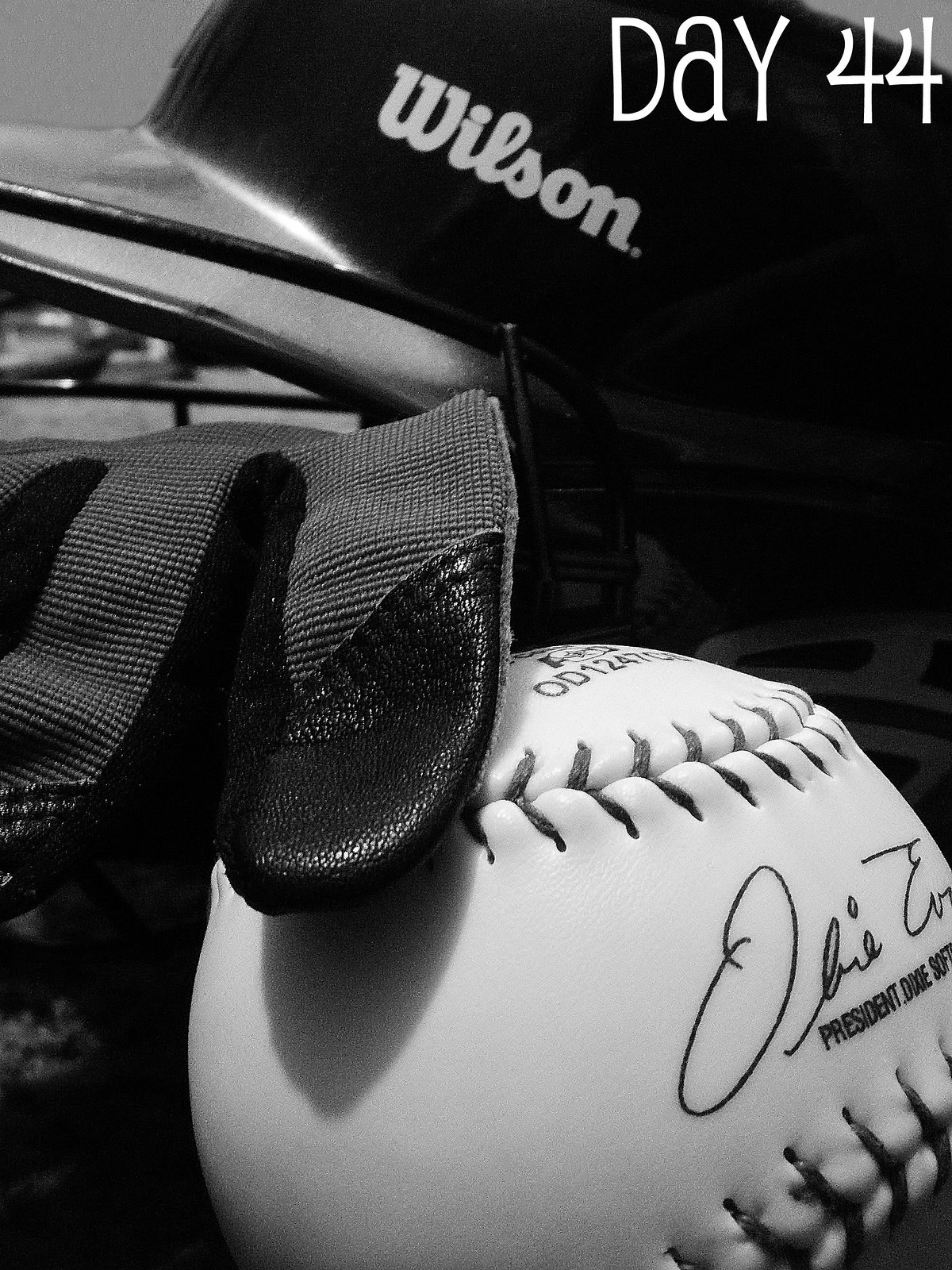This black-and-white photograph showcases a close-up arrangement of baseball equipment. In the top right corner, white text reads "Day 44." Dominating the bottom part of the image is a white baseball, prominently featuring red seams and signed with the partially legible name "OB IE" followed by "President," and "Dixie Softball." Draped over the left side of the baseball is a pair of gloves, distinguished by black leather fingertips. Above the baseball and gloves, a black baseball cap with the brand name "Wilson" in bold white letters is positioned, adding a classic touch to the sports gear ensemble.